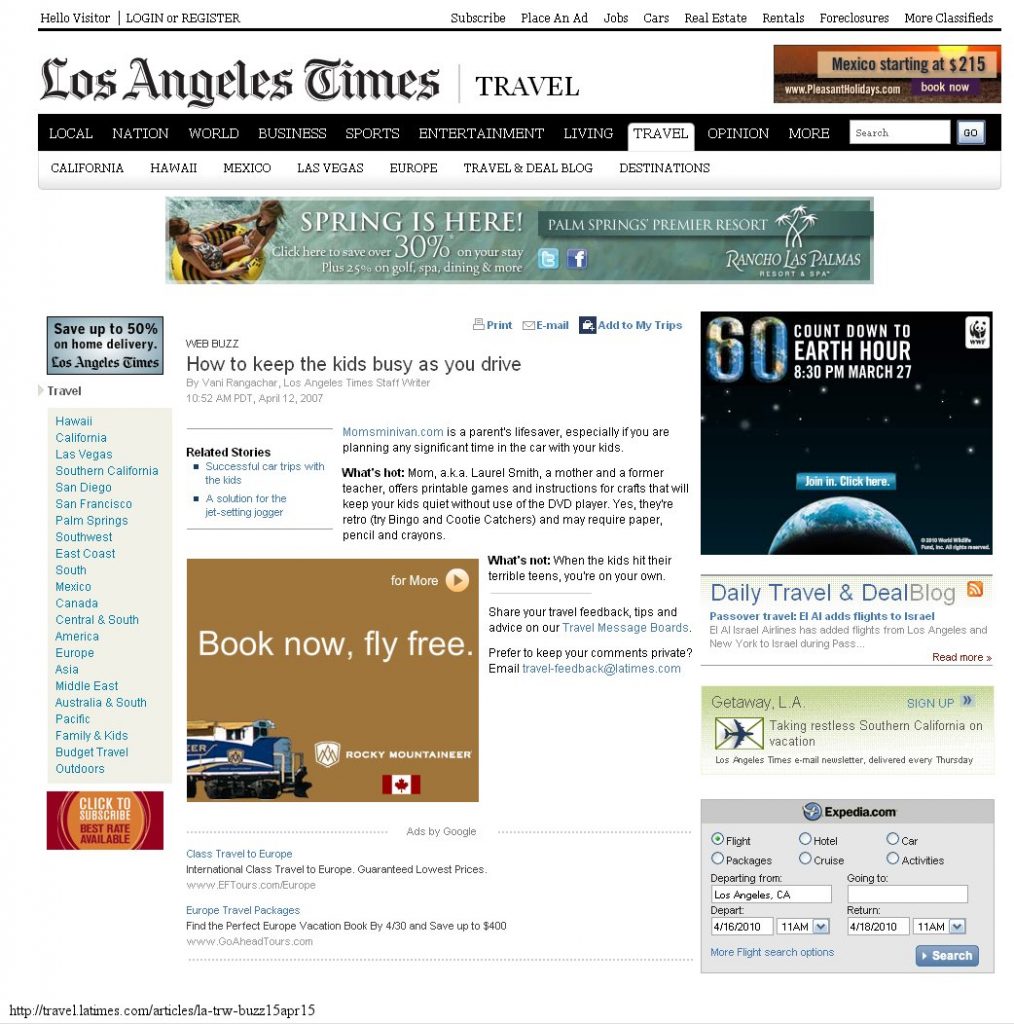A screenshot of the Los Angeles Times travel section is densely packed with various advertisements and links. The main focal point is an advertisement featuring people in a yellow floatation device in the water, accompanied by the text, "Spring is here, save 30% at Palm Springs Premier Resort." Other prominent ads and notices include offers such as "Save up to 50% on home delivery," "Book now, fly free," and a 60-day countdown to Earth Hour on March 27th at 8:30 PM, encouraging readers to join in.

Additional travel destinations and services are highlighted, such as California, Hawaii, Mexico, Las Vegas, Europe, and various travel and deal blogs. The page also features numerous links for subscribing to the newspaper, placing ads, finding jobs, cars, real estate, rentals, and more classified sections.

Prominent advertisers include Expedia.com and Google, offering deals like class travel to Europe and Europe travel packages. The high volume of advertisements overshadows the news content, suggesting a significant commercial influence in the section.